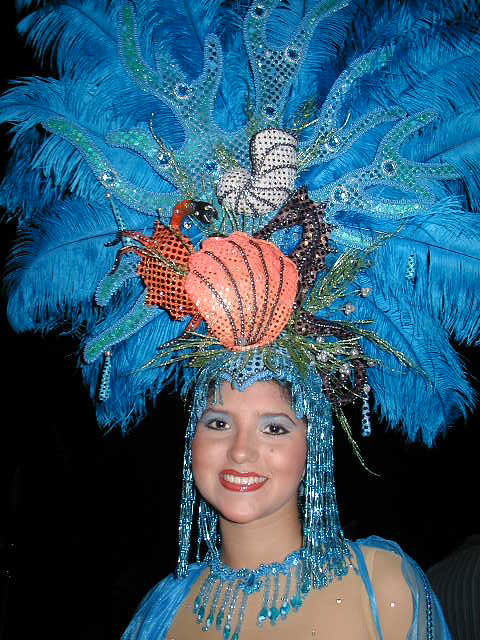The photograph features a young woman, potentially of Hispanic descent, adorned in a striking blue dress and an extraordinarily elaborate headdress that exudes an aquatic theme. The headdress starts with what appears to be a cap, from which purplish or blue fronds cascade down to her collarbone, mimicking hair. Rising from this cap is a magnificent corona of feathers that radiate circularly, forming a grand halo of tall, blue plumes.

Interwoven within this feathered halo is an intricate frame resembling elongated coral branches, enhancing the maritime motif. Nestled in the centerpiece are a variety of oceanic elements, including a crab, seashells, a seahorse, and entwined green seaweed. Complementing her ensemble, the woman wears striking blue eyeshadow and vivid red lipstick, with hints of her black hair peeking through the headpiece. This detailed costume piece transforms her into a mesmerizing vision of the sea.